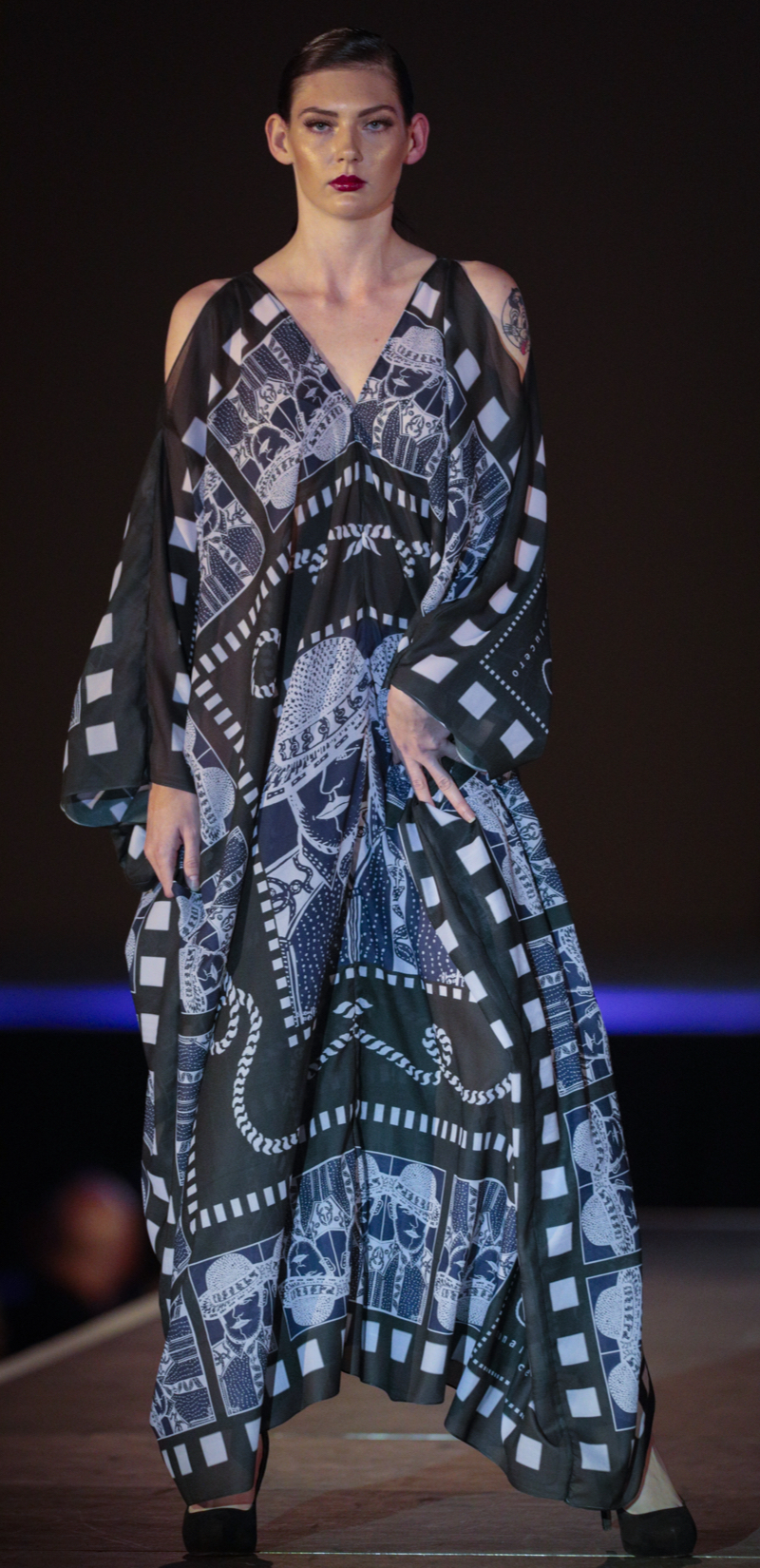The image features a tall female model walking down a black runway, wearing a long, baggy, black and blue dress. The dress is adorned with intricate, African-inspired, comic book-style designs, including a man's upper body and face with a flat hat, and a line of squares and additional male portraits along the bottom and sides. The dress has a V-neck, exposing the model's neck and upper chest, and shoulder cutouts, along with long sleeves that extend to her wrists. The model’s stoic face is accentuated with red lipstick and bright blue eyes. She has short, slicked-back brown hair, almost resembling a male haircut, and bears a prominent tattoo of a kid's popsicle on her upper left arm. Her legs are slightly apart, and she wears black high heels. The background is predominantly black, with a blue luminescent line running horizontally just above her knees. A blurry patron’s head is visible to the left of the runway. The model’s expression is neutral, yet serious, adding to the dramatic presentation of the fashion show.